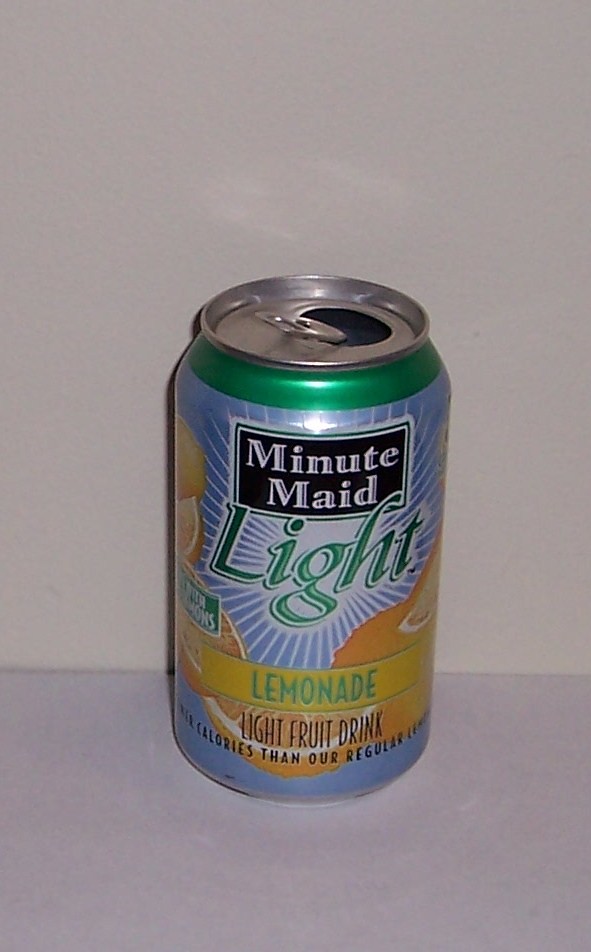The image showcases a tin can of Minute Maid Light Lemonade set against a backdrop featuring a light orchid wall and a darker orchid tabletop. The silver can has its lid popped open and is topped with a green rim. The can's label is a very light blue, adorned with a prominent black square that bears the Minute Maid logo in white letters. Below the logo, the word "Light" is prominently displayed in large, green letters, accompanied by subtle white sun rays radiating from it. The label also features vibrant yellow lemons, emphasizing the lemonade flavor. Additionally, "Lemonade" is printed in green letters, and "Light Fruit Drink" is inscribed in black letters at the bottom of the label.